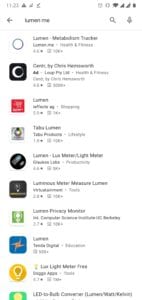This screen capture presents an out-of-focus image of a cell phone screen. At the top, the standard status bar displays the time as 11:21, alongside icons for battery life and other essential notifications. Below the status bar, the main portion of the screen contains a grid of app icons and their respective names, although most details are difficult to discern due to the blurriness of the image.

On the left side of the screen, a column features app icons, though their unclear nature makes it hard to identify specific apps. A variety of colors are visible among the icons, including a red square, a black circle, a blue square, and a yellow circle with what appears to be a lightbulb symbol. Despite the color cues, the icons remain indistinct.

To the right of each icon is a column likely listing the names and possibly the ratings of the apps, suggesting that this screen capture might originate from an app store or a similar interface. However, the text is mostly unreadable due to the lack of focus, rendering it impossible to fully comprehend the content.

Overall, while the image clearly indicates it is a capture from a cell phone, the significant blur obscures most of the specific details regarding the apps displayed. The intent behind this capture seems to be to showcase the apps present on the device, albeit unsuccessfully due to the poor image quality.